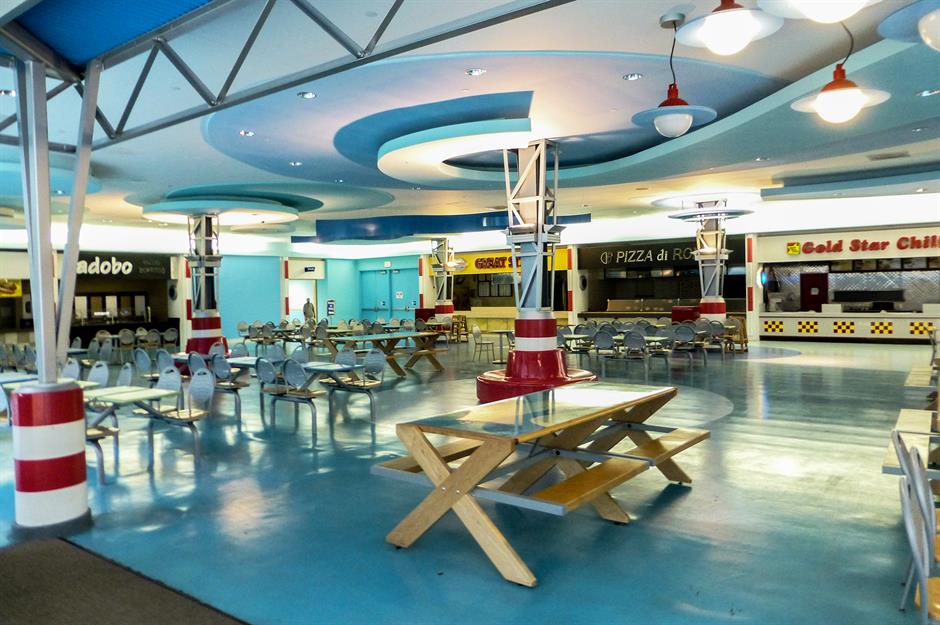The image depicts a seemingly closed, ocean-themed food court in a retro-style, modern mall, characterized by its various shades of blue. The ceiling, a light blue with intricate cutouts and swirls resembling the letter "J," features unique planetary lights with red and blue rings, resembling Jupiter. The aquamarine blue floor complements the decor, while blue-backed chairs, wooden benches with blue and brown accents, and several striped red and white pillars suggest an oceanic ambiance. Visible restaurants include Gold Star Chili, Pizza Di Rocco (partially obscured by a pillar), and Adobo. Additional features include a couple of picnic-style tables and several benches. In the background, an individual can be seen walking in from a hallway, adding to the atmospheric depth of the scene.